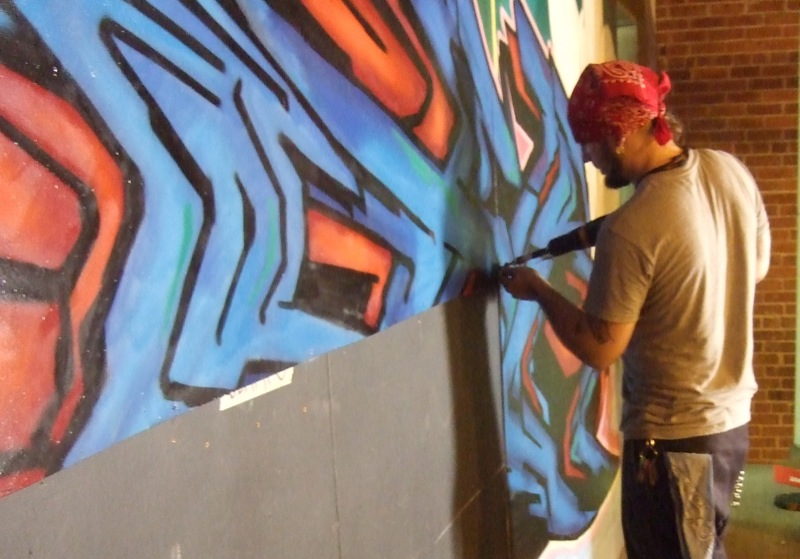This photograph captures a man in the process of assembling a mural on a wall, using a power drill to attach the final piece in a row of panels. The man, seen from a profile angle, is identifiable by his red bandana, a gray or beige shirt, and black or blue pants. He also carries a cloth tucked into his pocket and some keys hanging off his belt. Additionally, he sports a bit of a beard. The mural itself features a blue and red design, reminiscent of graffiti art, divided into several panels. The incomplete mural shows a section missing two pieces, revealing a grey background behind. Surrounding the mural is a standard brick wall, suggesting the activity might be taking place outside. The graffiti design includes blue lines intertwined with black scribbles, and red sections similarly embellished with black doodles, hinting at an old-school graffiti style.